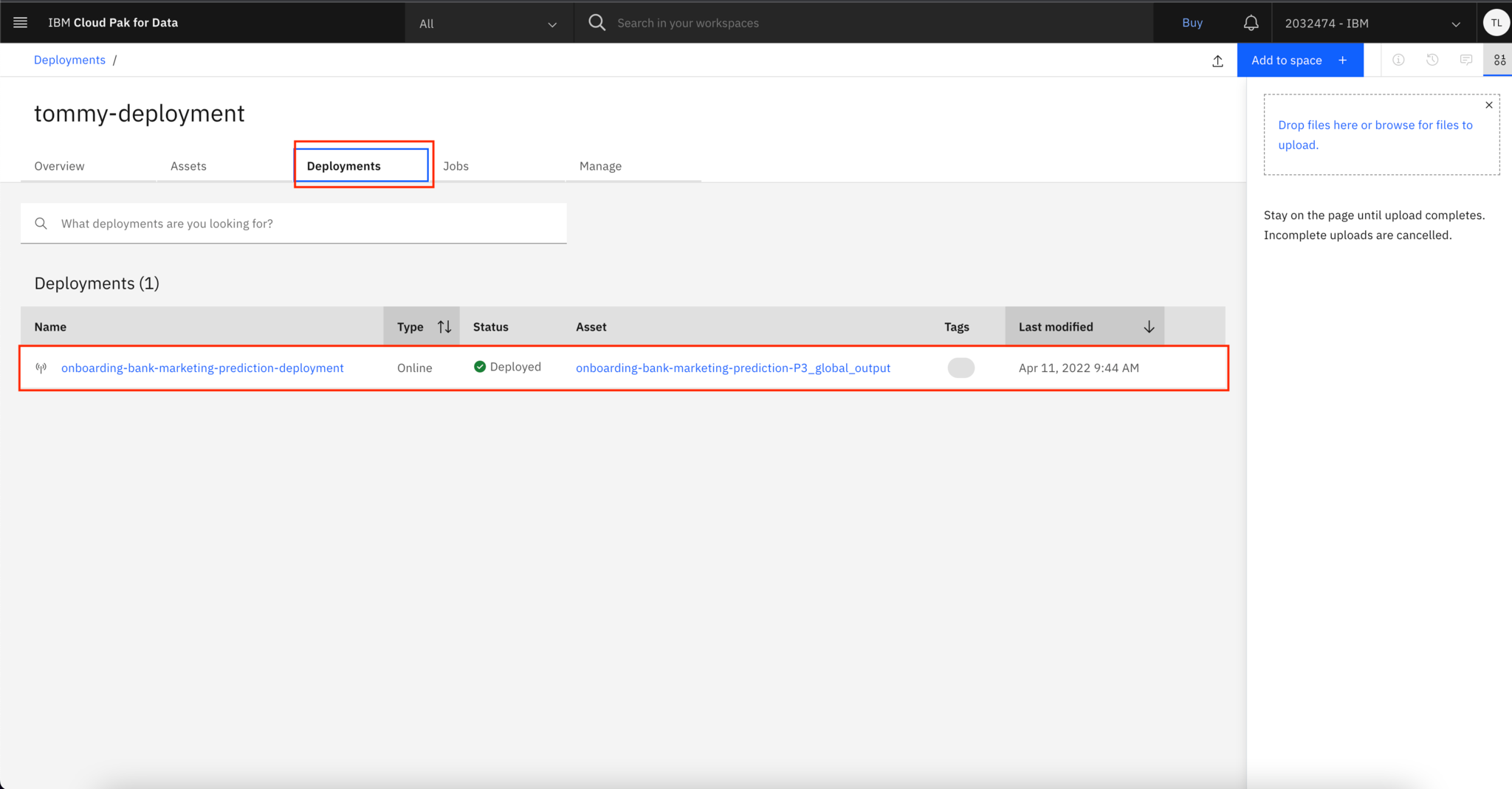The image is a screenshot of an online program taken from a computer screen. At the very top, there is a black navigation bar. On the left side of this bar, the text reads "IBM Cloud Pak for Data." On the right side, additional elements are displayed: a "Buy" button, a bell icon, a number labeled "2032474-IBM," and a white circle containing the letters "TL."

Below the black bar is a blue rectangular button labeled "Add to Space." Continuing downward, there is a box that provides the option to "Drop files here or browse for files to upload." To the left of this box, there is a section labeled "Deployments," followed by a subsection titled "Tommy Deployment."

The interface is divided into several tabs, including "Overview," "Assets," "Deployments," "Jobs," and "Manage." The "Deployments" tab is highlighted with a red and blue border. Directly under the highlighted tab is a search bar with placeholder text that reads "What deployments are you looking for?" Beneath this, there is another header labeled "Deployments (1)."

In the section below, there is a detailed box with the following information:
- **Name**: onboarding-bank-marketing-prediction-deployment
- **Type**: Online
- **Status**: Deployed
- **Asset Tags**
- **Last Modified**: [time and date]